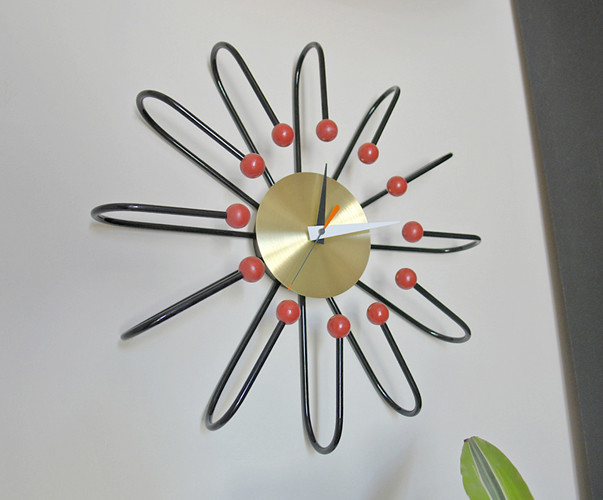This vibrant, color photograph captures a modern interior scene, focusing on a striking wall clock that serves as the centerpiece of the room. The clock features a small, round, flat gold disc at its center, from which the clock's hands emerge. The hour hand is black, the minute hand is white, and the second hand is distinctive with a thin form ending in a vivid orange tip. The time displayed on the clock is approximately 12:20.

Radiating from the gold disc, numerous black rods extend outward in a circular pattern. These rods are arranged meticulously, curving back towards the center and each ending with a small red knob. This intricate arrangement gives the clock a dynamic, floral appearance, reminiscent of a modern art piece made from metal. The careful design of the rods, paired with the color contrast of the hands, ensures that the clock is both functional and an eye-catching decorative element within the home.